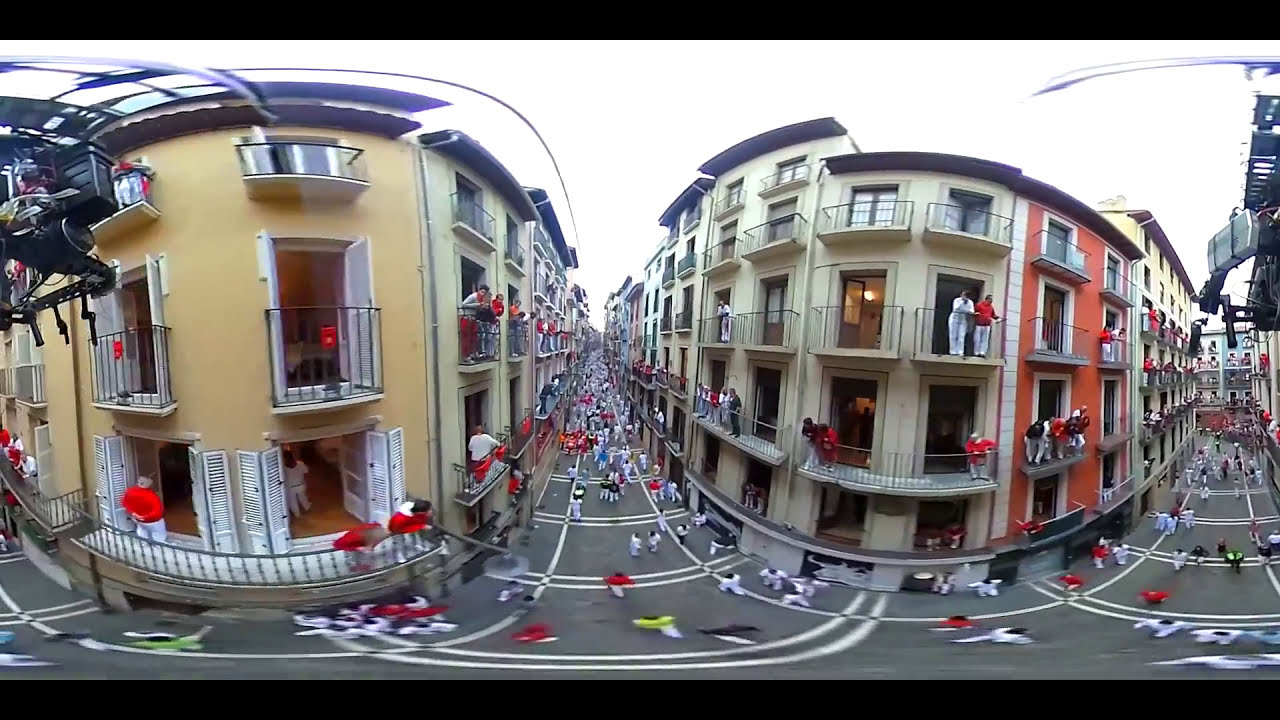The image is a vibrant scene of the Running of the Bulls festival, likely in Madrid, Spain, captured with a fisheye lens that slightly distorts the perspective. The city street runs horizontally across the bottom and extends upward through the center, branching off to the left and right. The scene is bustling with numerous people dressed predominantly in red and white shirts, running and walking down the street, which is flanked by two three-story apartment buildings. These buildings, positioned almost centrally in the image, feature balconies from which more people lean over metal railings to observe the excitement below. The image is rich with colors—white, yellow, black, red, green, blue, tan, and orange—despite the lack of any text. The outdoor setting, bathed in daylight, underscores a festive atmosphere in a residential area. Details like the curving buildings and the positioning of objects hint at a wide-angle lens addition to some camera equipment visible at the edges of the image, enhancing the overall dynamic quality of the photograph.